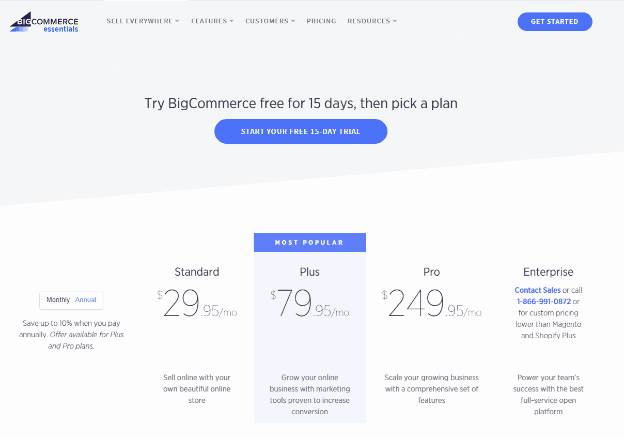This is a detailed screenshot of the BigCommerceEssentials website, showcasing its clean and functional design. The webpage is divided horizontally, with a grey top half and a white bottom half. In the top left corner, the BigCommerceEssentials logo is prominently displayed. To the right of the logo, there are navigation categories listed as "Everywhere," "Features," "Customers," "Pricing," and "Resources." On the far right side of the top navigation bar, a noticeable blue button invites users to "Get Started."

Centered at the top of the screen, a promotional banner encourages visitors to "Try BigCommerce free for 15 days and then pick a plan." Directly below this, a conspicuous blue bar further prompts users to "Start your free 15-day trial."

The main section below these prompts displays the subscription options in a clear and organized manner. In the bottom left corner of this section, there is an option to choose between "Monthly" or "Annual" billing, with the "Annual" option currently selected, offering a saving of up to 10% when paid annually.

Three main pricing packages are listed prominently with large, bold numbers:
1. **Standard** at $29.95 per month.
2. **Plus** at $79.95 per month, highlighted in a blue box with a "Most Popular" label above it.
3. **Pro** at $249.95 per month.

On the far right, there is an "Enterprise" option, which advises potential customers to "Contact Sales" or call a provided number for custom pricing. The detailed layout and inviting calls-to-action create a user-friendly experience, clearly presenting the offerings of BigCommerceEssentials.